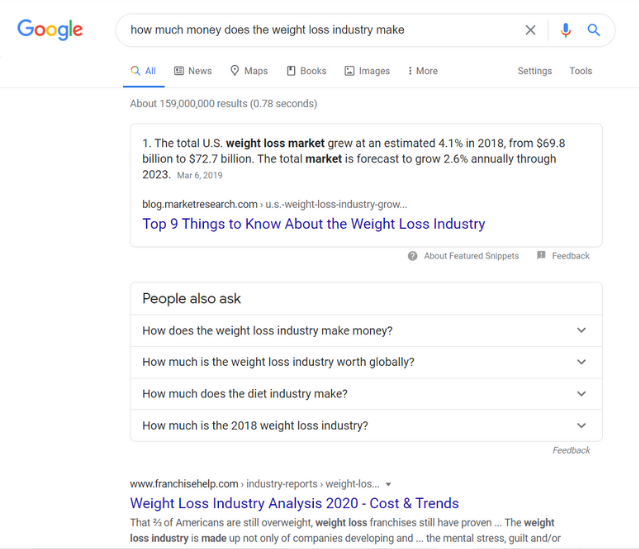The image displays the results of a Google search, with the Google logo prominently featured in the upper left-hand corner. The search query entered in the field reads, "How much money does the weight loss industry make?" To the right of the search field are the 'X' close button, a microphone icon, and a magnifying glass icon for voice and text search functionalities respectively.

Below the search bar, the interface shows multiple filter options including "All," "News," "Maps," "Books," "Images," "More," "Settings," and "Tools," with "All" currently selected. A total of 159 million results are generated in 0.78 seconds.

The first snippet highlights that the U.S. weight loss market grew by an estimated 4.1% in 2018, increasing from $69.8 billion to $72.7 billion. The total market is forecasted to continue growing at a rate of 2.6% annually through 2023, according to blogmarketresearch.com. One of the top search results is titled "Top Nine Things to Know About the Weight Loss Industry."

The “People also ask” section presents related questions in black text, such as "How does the weight loss industry make money?”, “How much is the weight loss industry worth globally?”, “How much does the diet industry make?”, and “How much was the 2018 weight loss industry worth?” Below this section is another result labeled "Weight Loss Industry Analysis: 2020 Costs and Trends," from thefranchisehelp.com.

The page is predominantly text, with links in blue and the majority of the other text in black, including the interactive "People also ask" section, which although clickable, remains in black text.